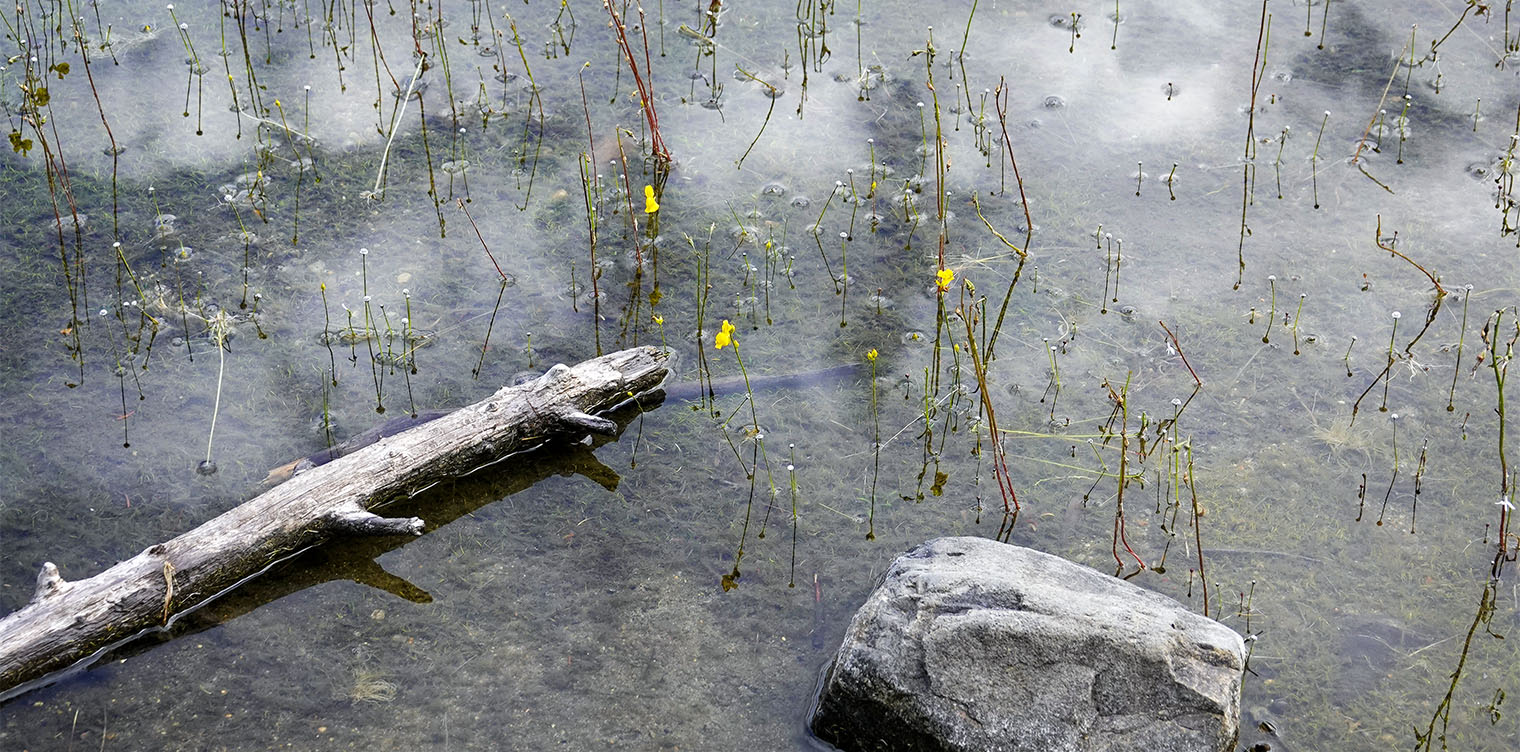The photograph captures a serene yet desolate marshland scene, predominantly in muted tones despite being in color. The water, extremely shallow and clear enough to reveal subaquatic plant life and patches of algae, holds a murky surface, creating a slightly misty ambiance that suggests early morning. Scattered across the scene are numerous skeletal plants, their bare stems piercing the water's surface, punctuated occasionally by delicate yellow and white flowers. Dominating the left side is a bleached, barren log, devoid of leaves and branches, lying partly submerged. On the right, a substantial gray stone—possibly granite, marred with white splotches—juts out of the water. The photograph, oriented in a wide rectangle, artfully encapsulates the stillness and eerie beauty of this swampy landscape.